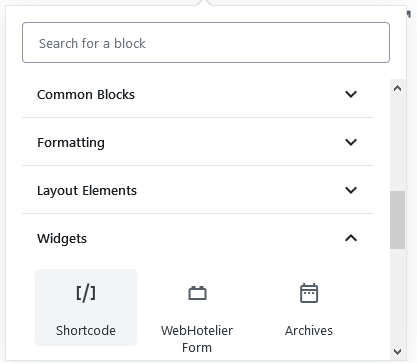The image features a user interface with a primary light gray background, overlaying a white section outlined with a light gray border. At the top of the white section, there's a search field with the placeholder text "Search for a block" in gray. Below the search field, several dropdown menus are displayed in a bold, dark gray font. 

The first dropdown menu reads "Common Blocks" with an arrowhead pointing downward to indicate it can be expanded. This is followed by a thin gray line acting as a divider. The next menu is labeled "Formatting," again accompanied by a downward-pointing arrowhead and a gray divider line. Below this, "Layout Elements" is listed, also with a downward-pointing arrowhead and a gray divider. The last dropdown menu is "Widgets," but this arrowhead is pointing upwards, signifying that it is expanded.

Within the expanded "Widgets" section, there are three options. The selected option on the left is highlighted with a gray square background, featuring an icon of two brackets with a forward slash in the middle and labeled "Shortcode." The center option displays a gray Lego block icon with the text "Web Hotelier Form" underneath. The option on the far right has a gray calendar icon and is labeled "Archives."

To the right of these options is a vertical scroll bar. The scroll bar's position is indicated by a dark gray segment in the middle of the bar, while the rest of the bar is light gray.